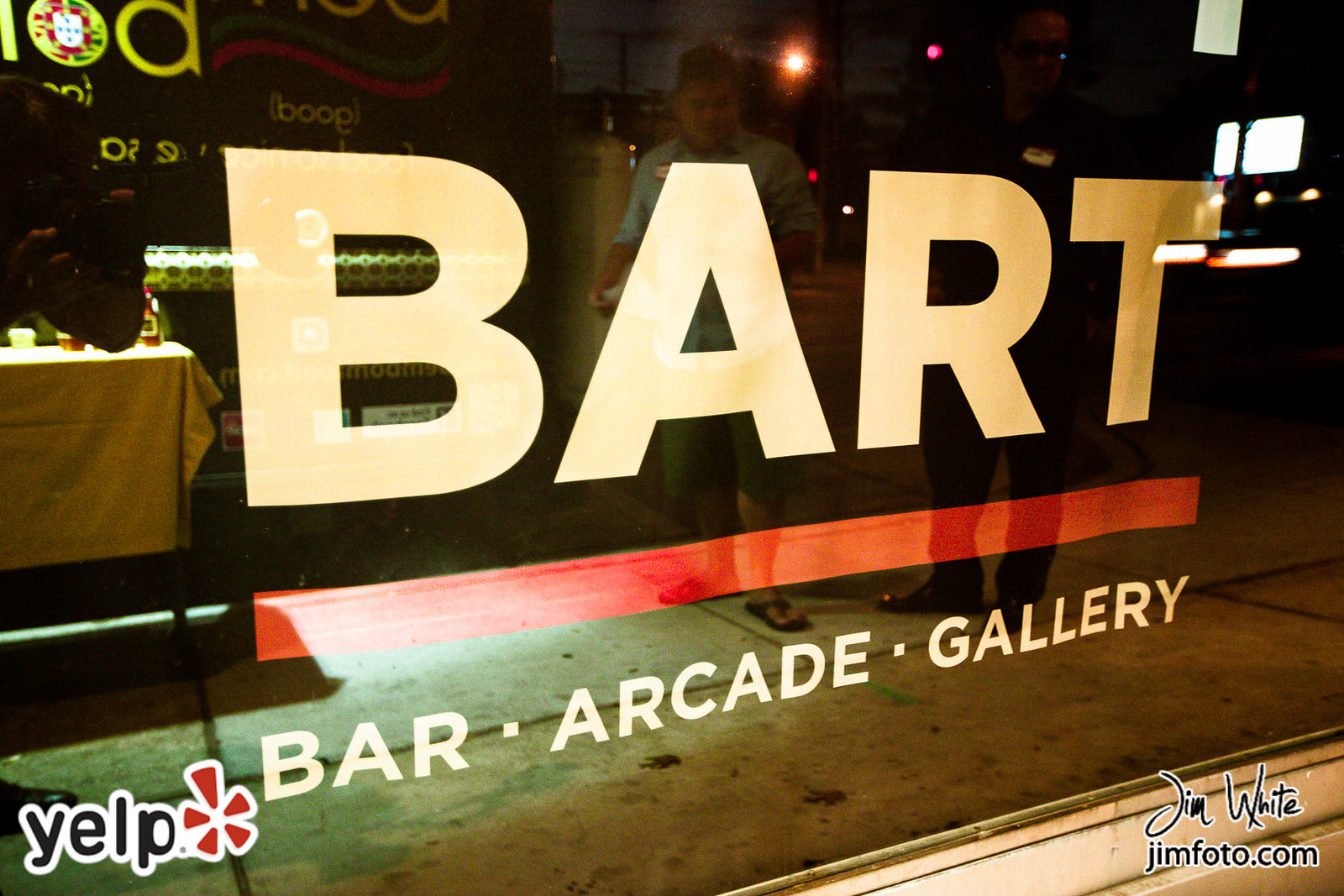The photograph captures the front window of a business named "Bart Bar Arcade Gallery," with the signage prominently displayed in white text. Below the name “BART,” a horizontal red line separates it from the description beneath: "Bar Arcade Gallery." Reflected in the window's glass are two people, presumably observing the sign. The window's glass is partially transparent, revealing the dim interior that hints at a table with a tablecloth to the left and a glowing white rectangle, likely an arcade game, in the background. Imposed at the bottom corner of the image, there is a black Yelp logo with white-bordered text reading "Y-E-L-P" and an adjacent red starburst symbol. The photograph is credited to Jim White, as indicated by the inscription in black cursive text reading “Jim White” and the accompanying normal text “jimphoto.com” in the bottom right corner.